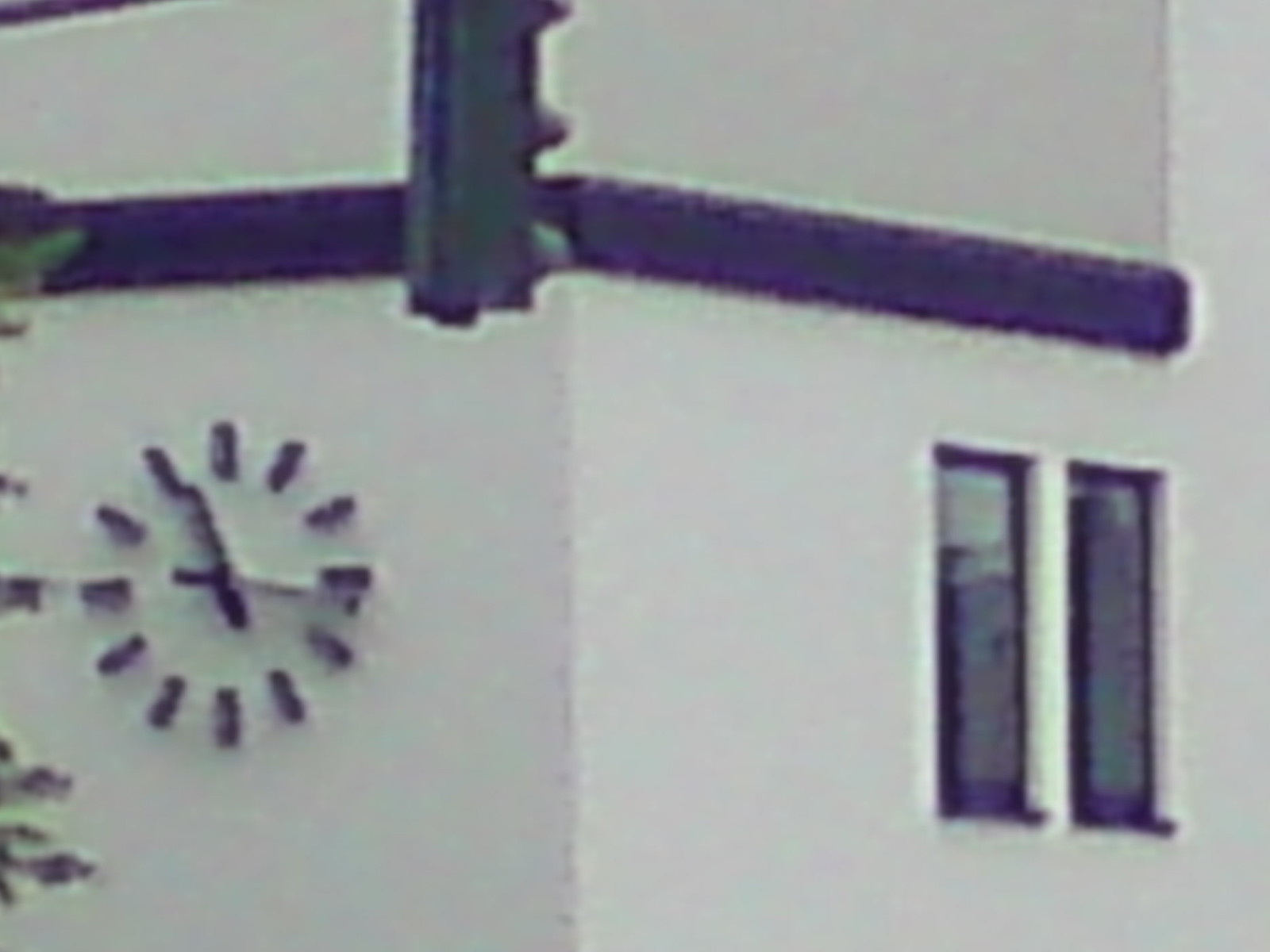The image depicts the exterior corner of a building with a white stucco or Adobe facade. A dark, royal purple line accentuates the top edge of the structure. On the left side, there is a stylized clock, outlined in purple without numerical markings, showing the time as approximately 11:16. To the right, two narrow, vertical windows are outlined in a similar purple hue. In the center top of the image, a black traffic light is suspended, facing right and presenting its rear side. On the left edge, green leaves from an adjacent tree are partially visible. The scene is rendered with a fine attention to detail, with contrasting elements of light gray and purple tones, suggesting a painting or drawing.